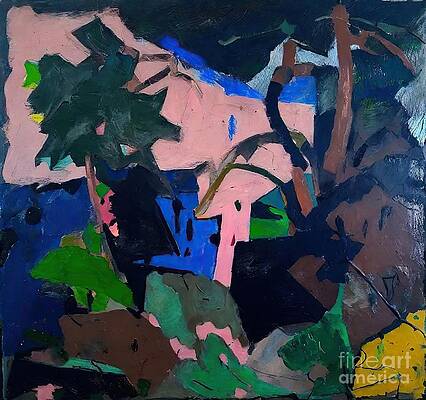This abstract oil painting features a dynamic composition with varied shapes and colors. Predominantly, it showcases blocky formations and shapes that suggest elements such as trees, buildings, and hills, all rendered in an abstract style. The right side is dominated by a brown color, which morphs into a tree-like structure with a green circular top. Blue shapes, hinting at buildings, can be seen in the background on the left. The foreground reveals green, dark green, and gray shapes resembling a hill, from which two black silhouettes emerge, also interpreted as tree forms with green tops. The top section of the painting has a substantial pink mass that contrasts with patches of medium and lighter blue, interspersed with black and brown areas. The bottom third of the artwork is rich with green, brown, and black hues, accented by a dark yellow shape in the bottom right corner that could be interpreted as a seashell. The painting is unsigned but features a watermark at the bottom right corner that reads "Fine Art America."